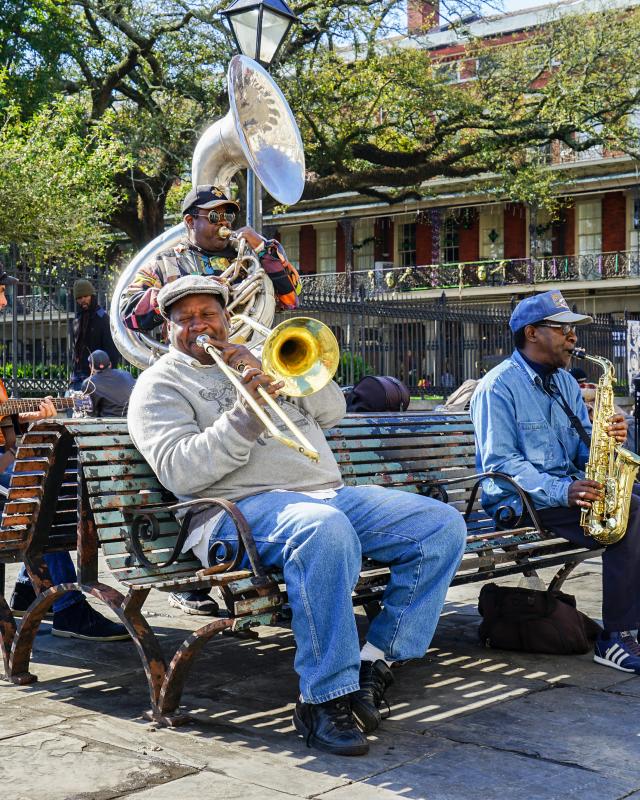This vibrant outdoor scene captures a lively brass band performance, likely set in a picturesque park in New Orleans, defined by its historical charm. Against the backdrop of a large, two-to-three-story red brick building adorned with white accents and a generous balcony, three African American musicians animate the space with their spirited play. The backdrop is partially cloaked by a sprawling tree, under a clear blue sky, adding to the relaxed, inviting atmosphere. 

Seated on a park bench are two musicians: the one on the left, a heavyset gentleman clad in blue jeans, dark shoes, a gray sweatshirt, and a gray snap cap, skillfully plays a trombone. Adjacent to him is a man sporting blue denim attire—a shirt and matching hat—dedicatedly playing a saxophone. Behind them, standing with commanding presence, another musician, donned in a vibrant, colorful sweater and a black baseball cap, energetically handles a large, gleaming silver tuba. 

Spectators mill about in the background, adding to the communal feel of the performance. The relaxed gathering and visible enjoyment among the musicians underscore a shared celebration of music in what appears to be a beloved communal space, resonant with the cultural heartbeat of New Orleans.